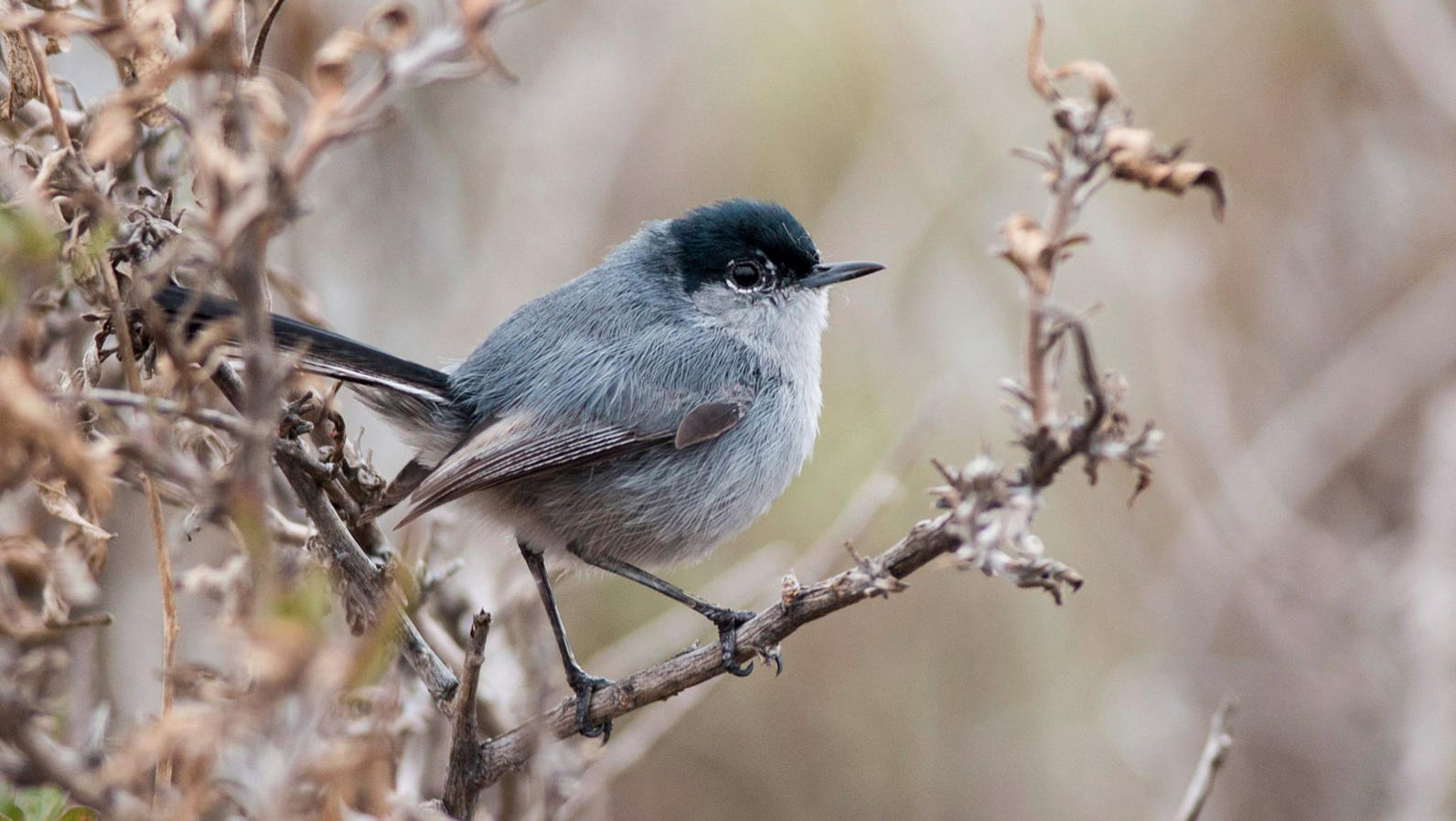The image showcases a small bird, primarily light gray with distinct black markings, perched on a barren, dry branch. Its head is a dark blue or black, blending seamlessly into pitch-black eyes and a small beak. The bird, presented in a detailed profile facing right, has a lighter gray belly, while its darker wings and tail showcase striking streaks of white. The background, a blur of brown hues with hints of green, emphasizes a winter or late fall setting with trees and foliage appearing lifeless and shriveled. The branch it grips with its thin legs is adorned with a few curled, dying leaves, enhancing the seasonal atmosphere captured in this close-up shot.